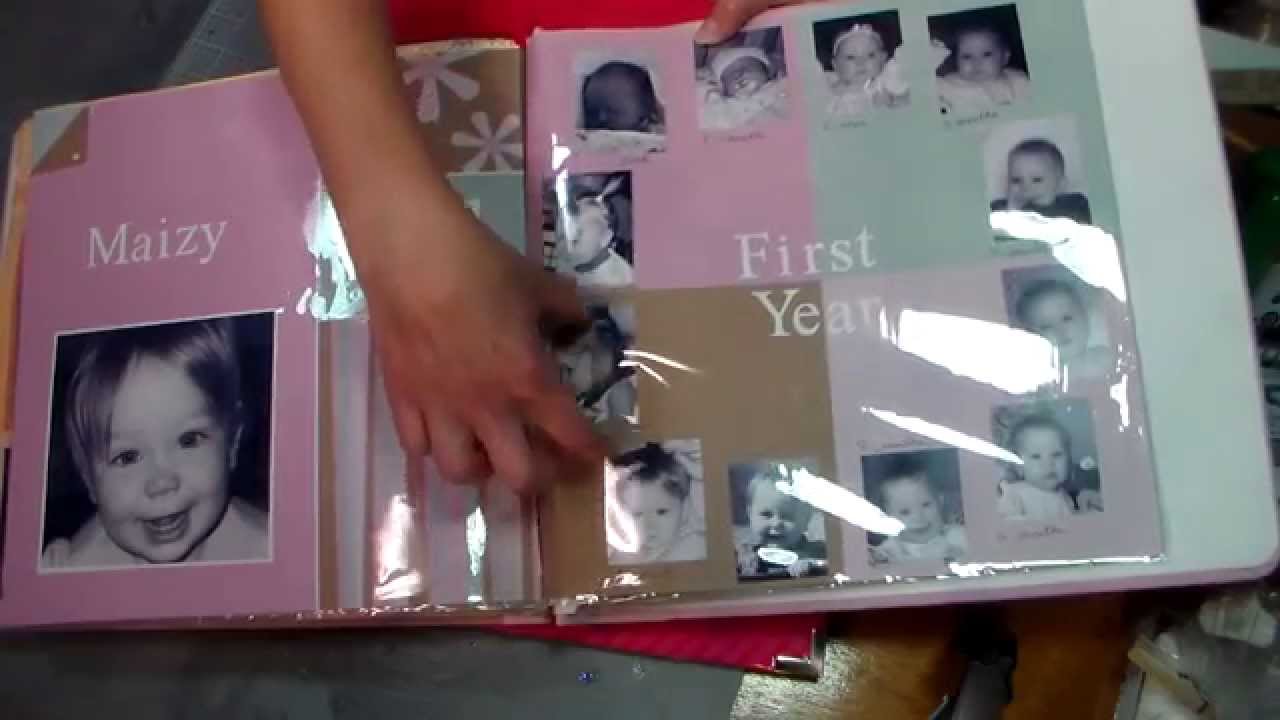The image showcases a baby book chronicling Maisie's first year. The book is adorned in pink and teal hues, featuring a plastic-coated, reflective surface. A human hand and part of a forearm are visibly holding the book open. On the left page, against a pink background with floral and striped accents, the name "MAISY" is prominently displayed in large white text. Below the name is a black-and-white photograph of a smiling baby, occupying almost half the page. The right page, with a teal background, is dedicated to the words "First Year" written in white at the center. Surrounding this central title, black-and-white photos of Maisie at various stages of her first year form a circular pattern. The top left quadrant of the page is pink, the top right is teal, the bottom left is brown, and the bottom right is a lighter shade of pink. The different quadrants and colorful scrapbook-style details enhance the overall design of the first-year album.